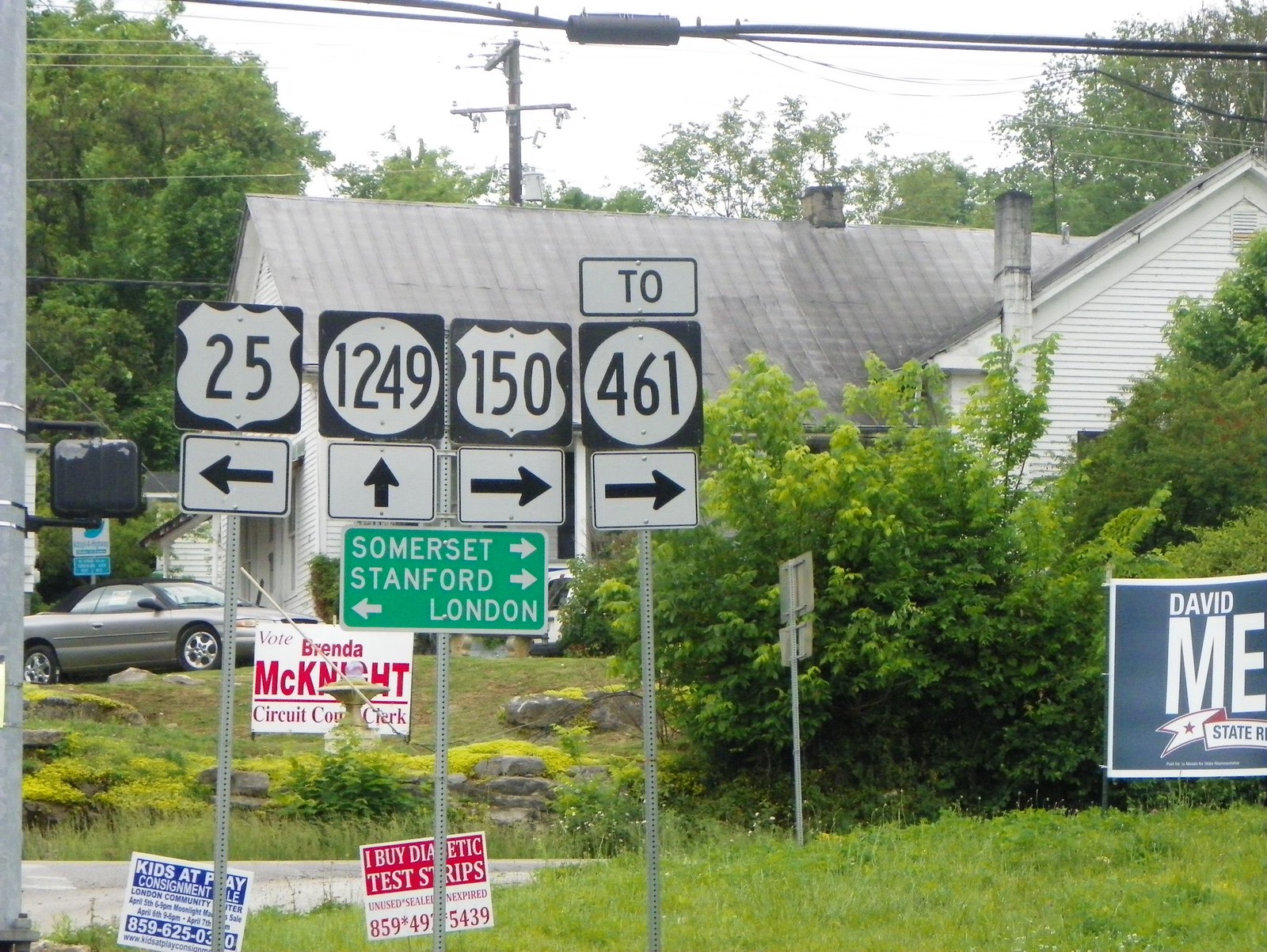The photograph captures an outdoor scene on an overcast day, with a distinctive white sky framed by trees on both the left and right sides of the image. Dominating the background is a white building with a gray roof, situated adjacent to a silver convertible car with a convertible top that appears in shades of gray and black.

In the foreground stands a cluster of street signs mounted on metal poles. The first on the left features a shield design with the number "25" and a left-pointing arrow beneath it. Next, a white circle marked "1249" with an upward-pointing arrow appears. Adjacent to it is another shield marked "150" with a black arrow pointing to the right. Further right, there's a sign with a white circle labeled "461" and a right-pointing arrow. Beneath these, a green rectangular sign indicates directions to nearby locations: "Somerset" and "Stanford" to the right and "London" to the left. 

Additionally, a political sign in the yard of the distant house supports Brenda McKnight for Circuit County Clerk, adding a touch of local electoral activity to the scene.